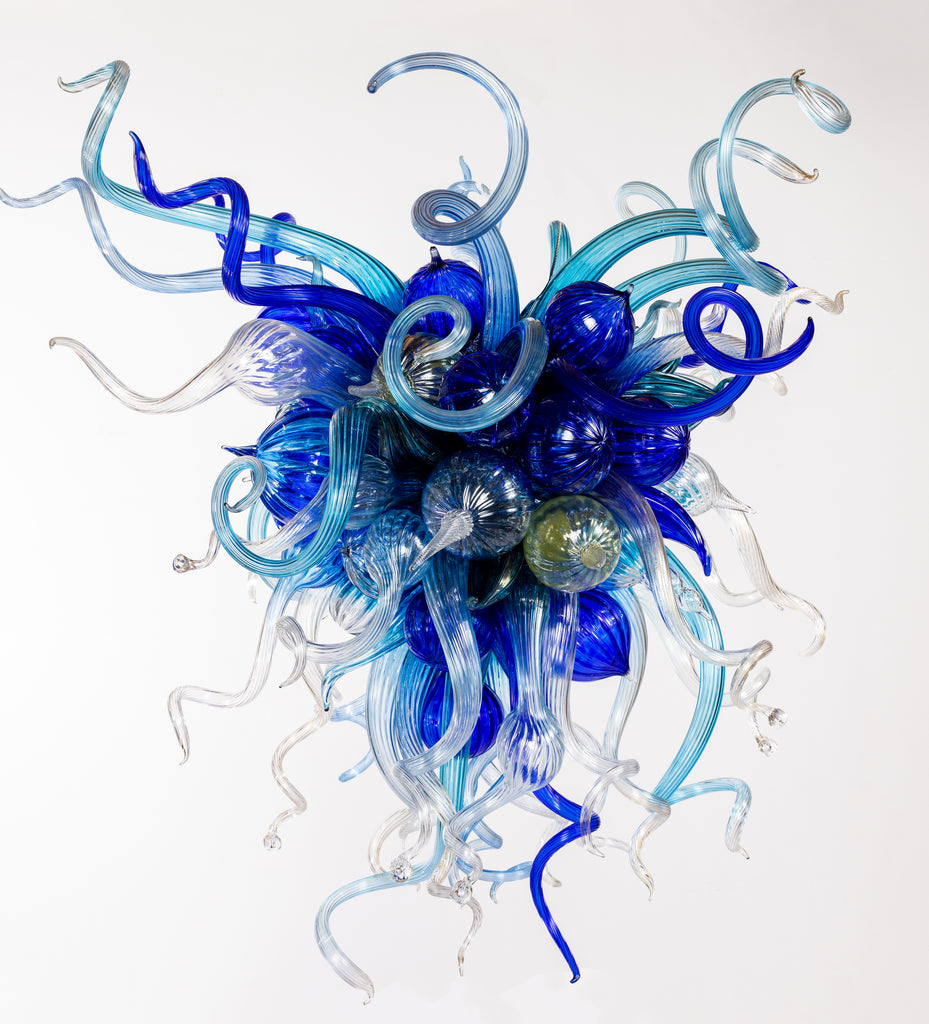This image showcases a mesmerizing piece of glass artwork, crafted in the distinctive style reminiscent of Dale Chihuly. Set against a stark white background, the centerpiece is an intricate glass sculpture that emanates a sense of dynamic energy and vivacity. At the heart of the artwork, a cluster of spherical blown glass globes in various shades of blue, ranging from deep navy to light aquamarine, some with clear or slightly translucent finishes, capture immediate attention. Intertwined among these spheres are numerous glass tendrils—akin to whimsical, elongated silly straws—that radiate outward in all directions. These tendrils vary in shape and size: some are long and sinuous, others shorter and more tightly curled, with the occasional one terminating in a pointed tip or a bulbous end, enhancing the overall texture of the piece. The tendrils and globes are predominantly blue, but sporadic touches of clear, white, and even a hint of yellow add an unexpected twist to the color palette. The seemingly chaotic arrangement of these elements evokes a vision of explosive movement, reminiscent of a starburst, or perhaps the frenzied serpentine locks of Medusa, infusing the artwork with an unmistakable sense of motion and life.